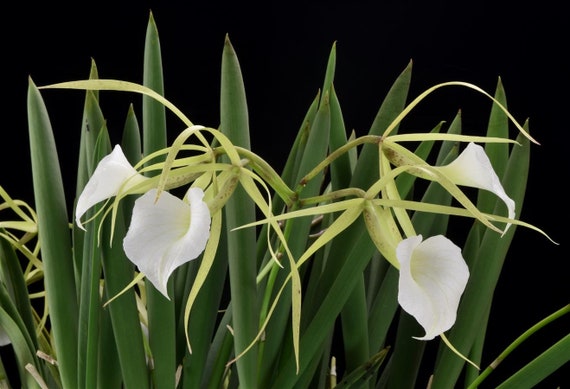The color photograph features four prominent white lily blossoms, each delicately bell-shaped and appearing soft to the touch. These blossoms stand out vividly against a stark, black matte background, creating a striking contrast. The lilies are surrounded by various types of foliage: tendril-like pale green stems emerge on the left, accompanied by long, sturdy, dark green leaves that resemble oversized blades of grass. These large, spear-shaped leaves are about two feet tall and stand uniformly straight, framing the elegant flowers. Additional light green leaves and unopened buds can also be observed, adding layers of depth and detail to the composition. The central white lilies remain the focal point, untouched by any signs of wilting, radiating freshness and purity.